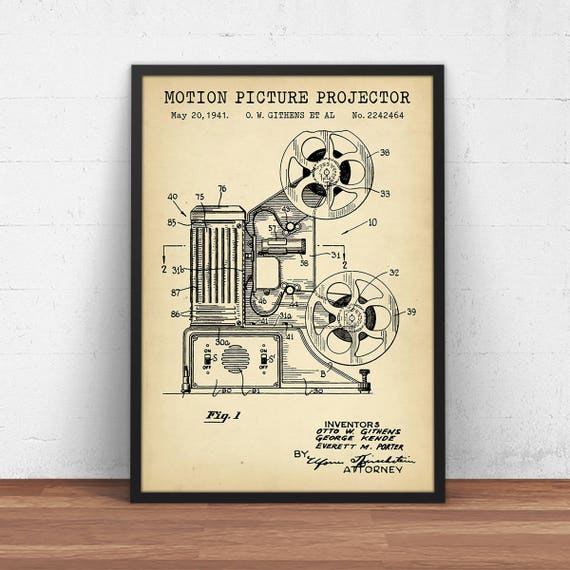The image showcases a framed poster leaning against a white brick wall, supported by a wooden floor. The poster, enclosed in a black frame, has a faded parchment color and features a detailed black-and-white diagram illustrating a motion picture projector. This diagram, which appears to be part of a patent application, is prominently labeled at the top with the title, "Motion Picture Projector, May 20th, 1941, O. W. Givens et al., number 2242464." The various components of the projector are marked with two-digit numbers ranging from 10 to 76. At the bottom left of the poster, "FIG-1" is clearly printed, while the bottom right lists the names of the inventors: Otto W. Givens, George Kendi, and Everett M. Porter. Additionally, a signature accompanied by the label "attorney" is present beneath the inventors' names. The entire scene is set against a minimalistic background, emphasizing the historical and technical significance of the patent.